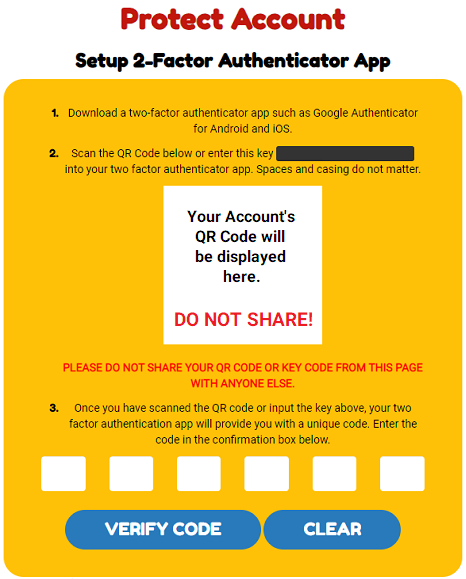**Screenshot of Two-Factor Authentication Setup Page**

The screenshot showcases a portion of a webpage dedicated to protecting a user's account by setting up two-factor authentication. The title "Protect Account" is prominently displayed in maroon bubble letters at the top.

Below the title, there's a large orange-yellow rectangle with rounded corners. This section contains detailed instructions highlighted with three bullet points:

1. **Download a Two-Factor Authentication App**:
   Users are instructed to download a two-factor authentication app such as Google Authenticator for both Android and iOS devices.

2. **Scan the QR Code**:
   Users are advised to scan the QR code provided, or manually enter the blacked-out key into their authentication app. The QR code area is represented by a white square with a placeholder text that reads "Your account's QR code will be displayed here." In bold red capital letters, users are cautioned "DO NOT SHARE."

   Additionally, a red warning text is displayed in the orange field: "PLEASE DO NOT SHARE YOUR QR CODE OR KEY CODE FROM THIS PAGE WITH ANYONE ELSE."

3. **Enter the Verification Code**:
   Once the QR code is scanned or the key is entered, the two-factor authentication app will generate a unique code. Users are prompted to enter this code into six white input fields aligned horizontally across almost the entire width of the orange space, with large spaces between them.

At the bottom of this section, two blue capsule-shaped buttons with white capital letters in bubble font are provided. The left button, which is wider, reads "VERIFY CODE," and the right button reads "CLEAR."